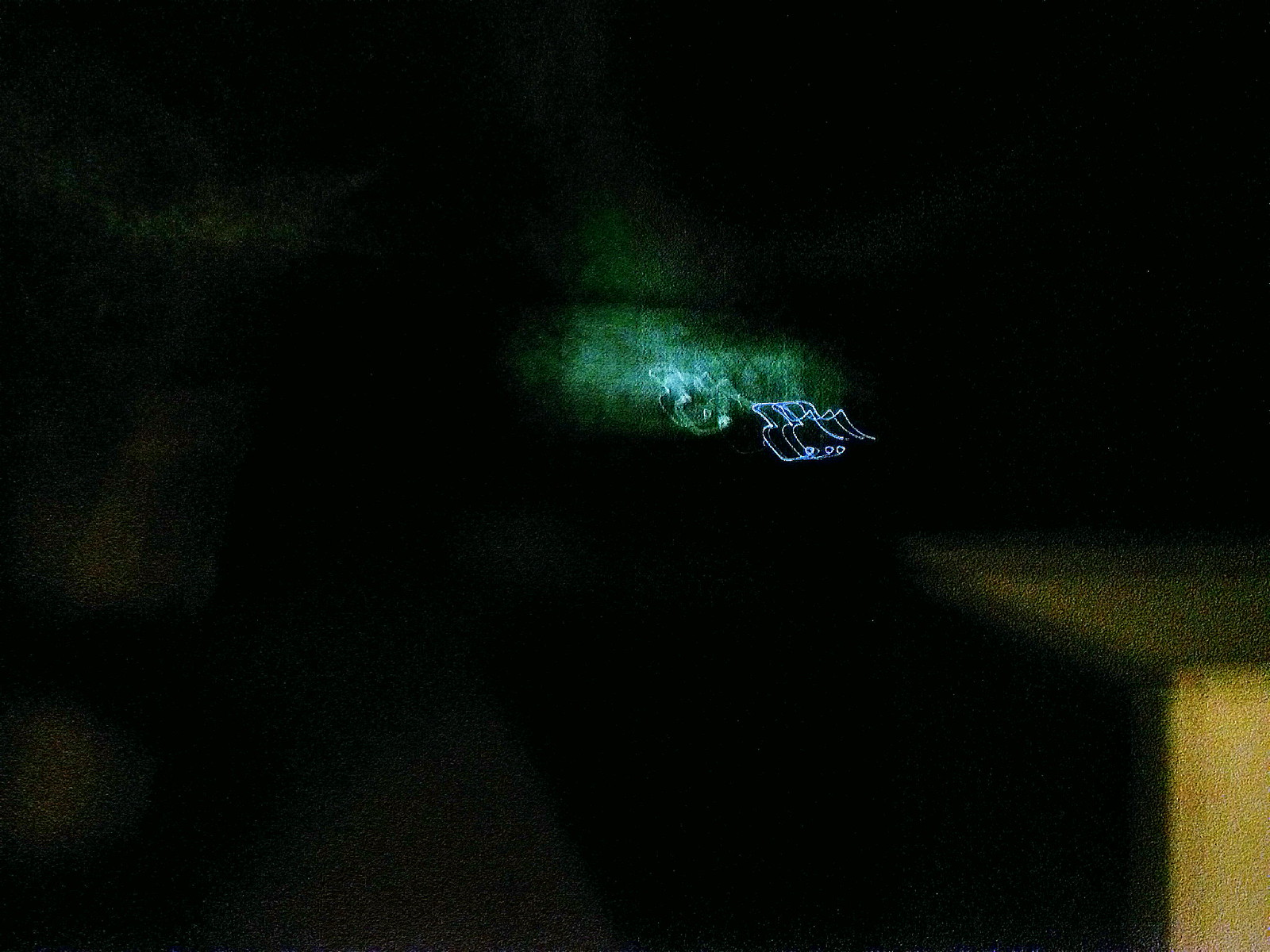A night-time photograph captures an abstract, enigmatic scene. The image is characterized by extreme blurriness, likely resulting from the camera's motion during the exposure. Dominating the composition is a mostly black canvas, suggesting the photo was taken in near-complete darkness. At the center, a faint, misty green light source emits a soft glow, adding an eerie ambiance to the image. Irregular, jagged blue squiggles emanate from this central light, cascading downward in rows, contributing to the surreal quality of the photograph. In the bottom right corner, a small, indistinct yellow box faintly emerges from the shadows, adding to the mystery and depth of the scene.